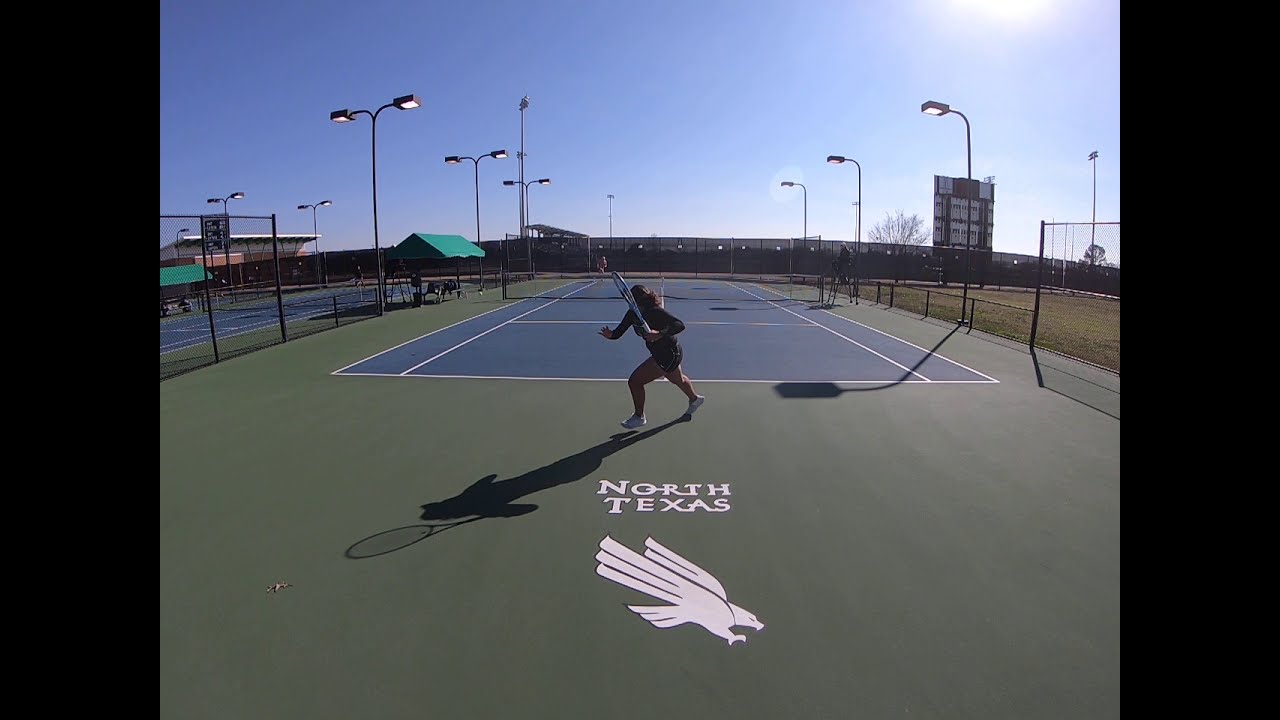The image depicts an outdoor tennis match set on a sunny, clear day with a bright blue sky. Central to the composition are two tennis players in the midst of a game on a blue court with white markings, encased by a surrounding green area. The player in the foreground, identifiable as a woman in shorts, is captured in a dynamic pose, seemingly rushing forward with a large silver tennis racket in her left hand, ready to swing or return a serve. She casts a long shadow across the court, suggesting the sun's bright presence in the top right corner. In the background, another player is visible, and an official oversees the match from the side.

Dominating the bottom of the image is a white logo with the words "North Texas" in an all-capital serif font, accompanied by an emblem depicting a flying falcon or eagle. To the left of the main court, a small green awning and a fence line are visible, beyond which lies another identical tennis court. The scene is also framed by vertical black stripes along the left and right sides of the wide horizontal rectangular shot, adding contrast to the vivid colors within the image: shades of green, blue, white, gray, and black.